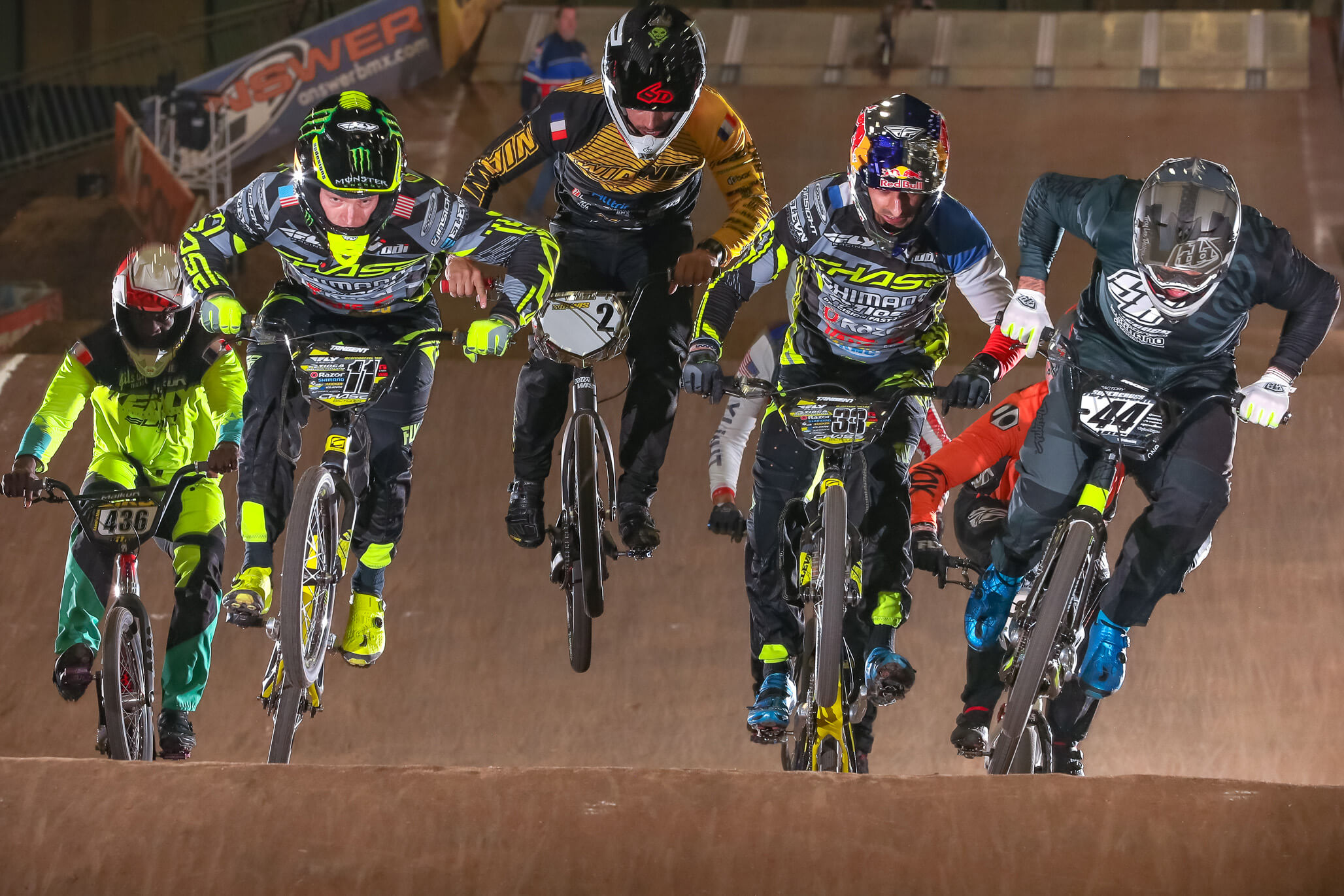The photograph captures an intense moment in a dirt bike race, featuring five riders navigating a dirt hill. The rider on the far right, number 44, leads the group in an all-black outfit. Next to him, number 33 sports a Red Bull helmet and a sponsor-laden jersey. The central rider, number 2, has just launched off a ramp, his bike airborne. He wears a light brown jersey paired with a dark helmet. Rider number 11, decked out in a black uniform with bright yellow trim, follows beside him. The final rider, number 436, lags slightly behind in an all-yellow outfit and a distinctive white and red helmet.

The track comprises brown dirt, featuring visible hills and ramps, including a long brown ramp in the background. On the left side of the image, there are several signs, one notably displaying the text "NSW ER" in orange and "our honest where? BMX.com" in white on a gray background. Each rider’s bike bears a distinct number on a white or colored background, enhancing their individual identifiability. The scene is energized by the riders' varied gear and national flags, including American, French, Estonian, and possibly Singaporean, adding an international flair to the competitive atmosphere.